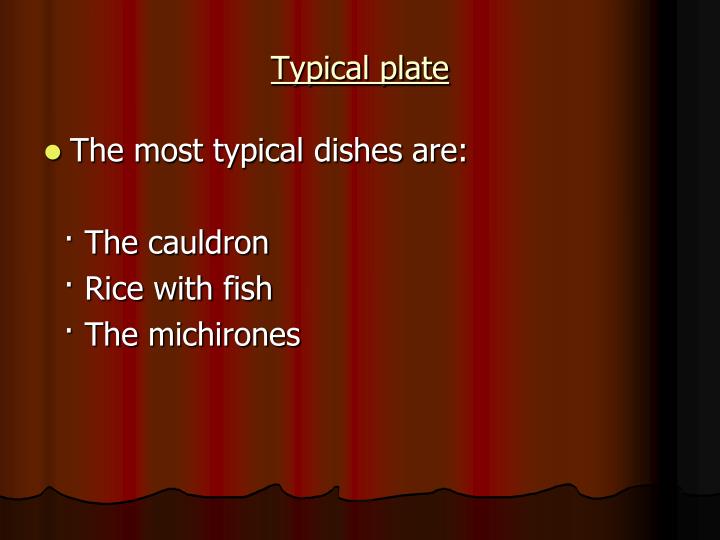The image is a rectangular PowerPoint slide designed to mimic a theatrical curtain with a color palette primarily in shades of orange to maroon-red. Vertical white lines run down the curtain background, which fades into black on the right-hand side. The bottom part of the slide features a scalloped edge meant to represent the top of the curtain and a stage floor in a slightly darker shade of maroon-red. At the top center of the slide, in bold, underlined white text, the title reads "Typical Plate." Below this, there's a large yellow bullet point followed by the text "The Most Typical Dishes Are:" with a colon. Below this statement are three square white bullet points, each listing a dish: "The Cauldron," "Rice with Fish," and "The Michirones." The text and layout emphasize the dish names, which are presented in a clear and concise manner.